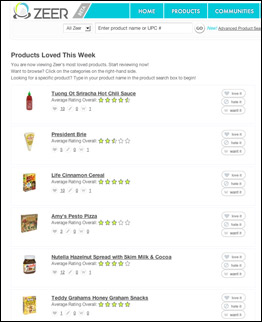On the homepage of the Zeer (Z-E-E-R) website, the company’s logo is prominently displayed in the upper left-hand corner in gray. The logo consists of a circular symbol, combining shades of teal and light gray, with two delicate gray swirls emerging from the bottom. A teal navigation bar sits above, segmented for easy access, featuring tabs labeled "Home," "Products," and "Communities," while the first section is notably empty. 

Beneath the navigation bar lies a search field, allowing users to search by product name or UPC number. Directly under this, a headline proclaims “Products Love This Week,” accompanied by a brief write-up. Below the write-up is a list of featured products, albeit with very small text that makes the descriptions difficult to decipher. 

The images of the products are clearer: one appears to be a bottle of some sort, another is a box of "Life" cinnamon cereal, and there's also a container of Nutella visible. Other listed items include something by "President," an "Amy's something pizza," and "Teddy Grahams." Each product is accompanied by green star ratings. On the right side of each product listing, there are three small boxes with indiscernible text due to the tiny font size used.